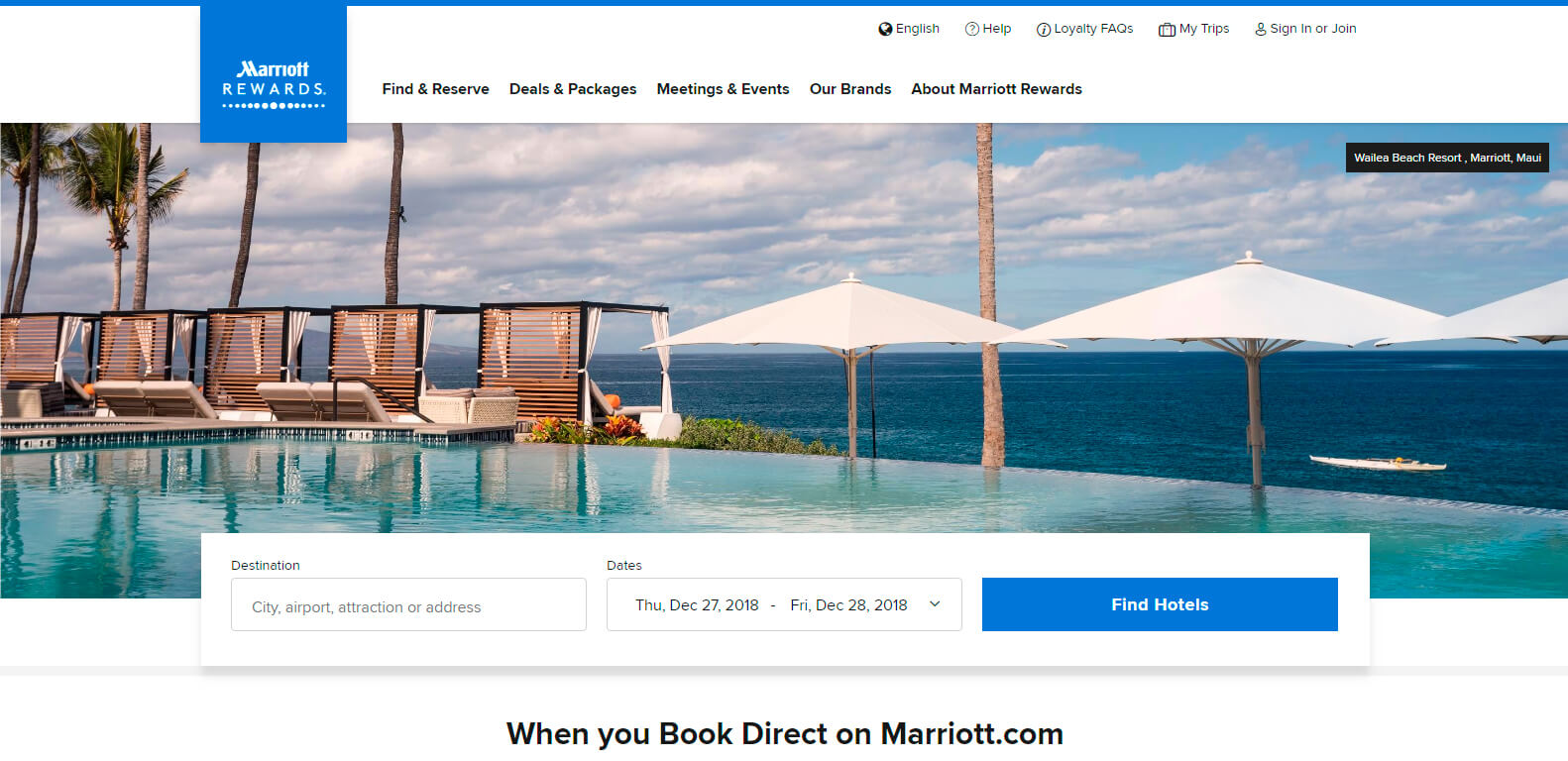This image is a screenshot from the Marriott Rewards Hotels website, specifically showcasing the Wiley Beach Resort Marriott. Dominating the center of the screenshot is a captivating photograph that spans almost the entire width of the display, featuring an inviting infinity-style swimming pool merging seamlessly with the open ocean in the background. The serene scene is enhanced by luxurious beach chairs and umbrellas arranged along the shoreline, and a person enjoying a kayak ride in the tranquil waters. The presence of palm trees suggests a location likely in Florida or California.

Below the image, there is a search bar where users can input their destination, city, airport, attraction, or address. Next to the search bar, date fields are already filled in with the text highlighted in darker black, indicating pre-selected dates of Thursday, December 27, 2018, and Friday, December 28, 2018. Adjacent to the date fields is a button labeled "Hotels," styled in a non-highlighted blue with white text, indicating it is interactive but not currently selected.

At the top of the webpage, there are navigation options for "Find & Reserve," "Deals & Packages," "Meetings & Events," "Our Brands," and "About Marriott Rewards." In smaller text at the very top, there are options for "English," "Help," "Loyalty," "FAQs," "My Trips," and "Sign In or Join." In the top right-hand corner of the image, the text "Wiley Beach Resort Marriott" is subtly displayed, tying the picturesque scene to its luxurious location.